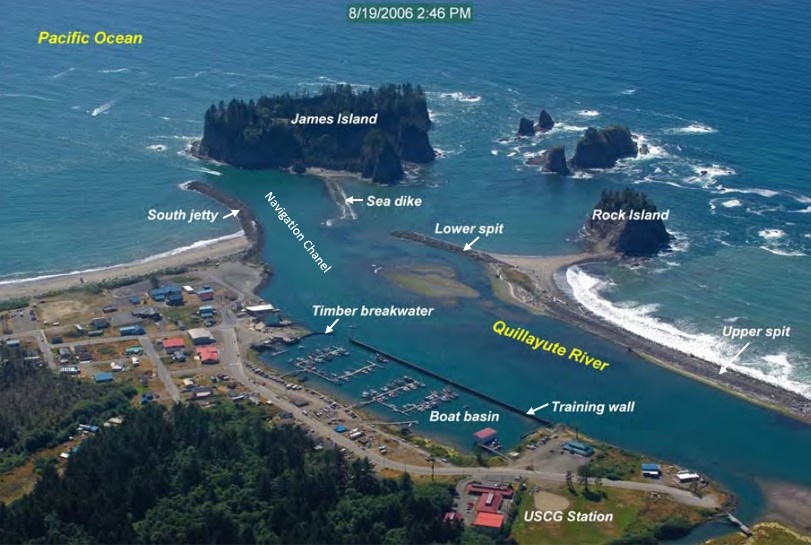This detailed aerial photograph, taken on August 19, 2006, at 2:46 PM, is annotated to highlight various geographic and man-made features near a large body of water labeled in yellow as the Pacific Ocean. In the upper left, James Island is prominently displayed, separated from the beach by a south jetty that creates a navigation channel. Below James Island, Rock Island is connected to the upper spit by a gravel or sand path, with smaller rocks situated to the right. The Quillayute River, correctly spelled out in yellow, flows nearby and opens up into a marina-like area known as the boat basin, which is separated from the river by a training wall. Additional labeled features include the Sea Dyke, Timber Breakwater, and South Jetty, as well as a USCG Station located toward the bottom left, near several buildings, roads (both asphalt and dirt), and trees. The upper left quadrant of the image is also marked with these detailed annotations in yellow, providing a comprehensive guide to the landscape and infrastructure.